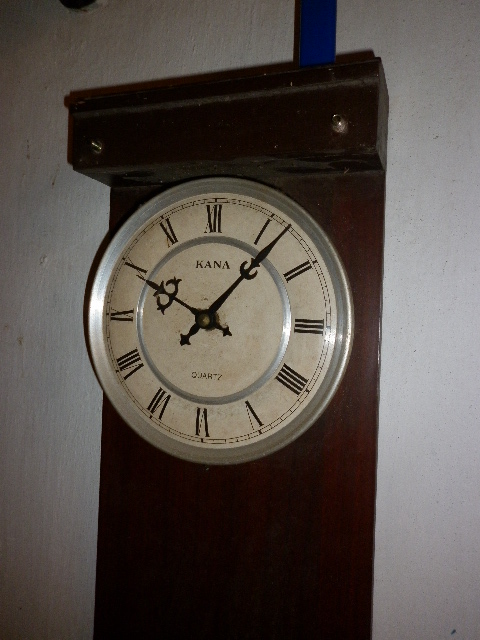The photograph captures an indoor scene featuring a sophisticated wall clock mounted on a white wall. The clock itself is circular with a polished silver border and an off-white face, displaying the time at 10:07. The Roman numerals, written in black, and the black ornate hour and minute hands stand out clearly. The clock is positioned on a rectangular piece of dark wood, likely mahogany, that serves as both a background and a partial frame. This wooden backing has a protruding shelf-like ornamentation at the top. Additionally, a small blue pipe extends out from the top right corner of this shelf. Below the Roman numeral XII, the brand name "KANA" is prominently displayed in black capital letters, while 'QUARTZ' is subtley inscribed just above the six o'clock position. The photograph is taken at a slight angle from the right, resulting in a minor glare at the three o'clock position on the clock face.